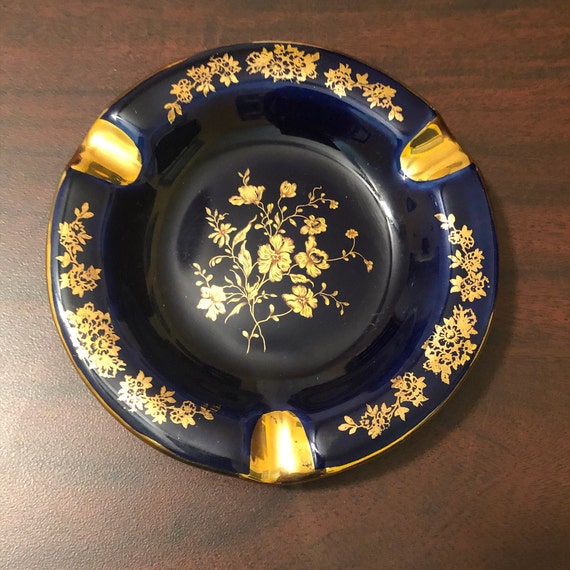The image showcases a close-up photograph of an ornate, shiny, dark blue ceramic ashtray resting on a brown wooden table with a dark grain pattern. The ashtray features a round, saucer-like shape with three notches designed for holding cigarettes or cigars; these notches are placed at the bottom, upper left, and upper right, and are painted gold. The edges of the ashtray are adorned with intricate gold floral patterns, which extend to the lip of the container. The center of the ashtray further displays an elaborate gold leaf and flower motif, characterized by thin stems and small leaves. Overall, the ashtray exudes a highly decorative and reflective quality, emphasized by its glossy finish and detailed gold accents.